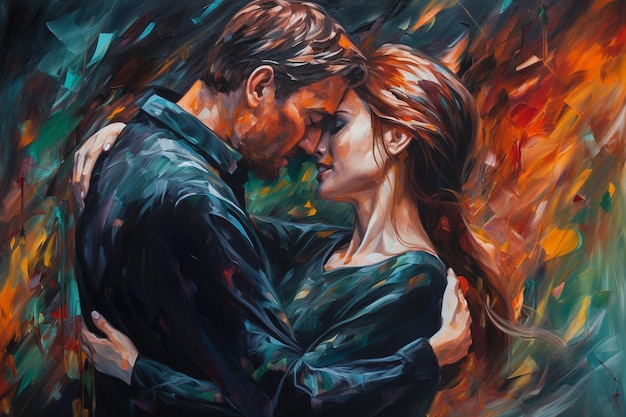In this romantic painting, a man and a woman are depicted with their noses nuzzling together, their arms tenderly wrapped around each other as they face one another, creating an intimate and heartfelt moment. The man, positioned on the left, has short brown hair, while the woman, on the right, has long flowing brown hair. Both of them seem to have their eyes closed, absorbed in the anticipation of a kiss. The background bursts with a blend of dark, autumn, and vibrant hues, including shades of orange, yellow, green, and blue, providing a rich and colorful backdrop to their embrace. The man is adorned in a dark, collared shirt that closely matches the dark v-neck shirt worn by the woman. Adding a touch of allure, the woman is highlighted with blue eye makeup, and her slightly open mouth reveals a glimpse of her front teeth, further enhancing the intimate atmosphere of the scene.